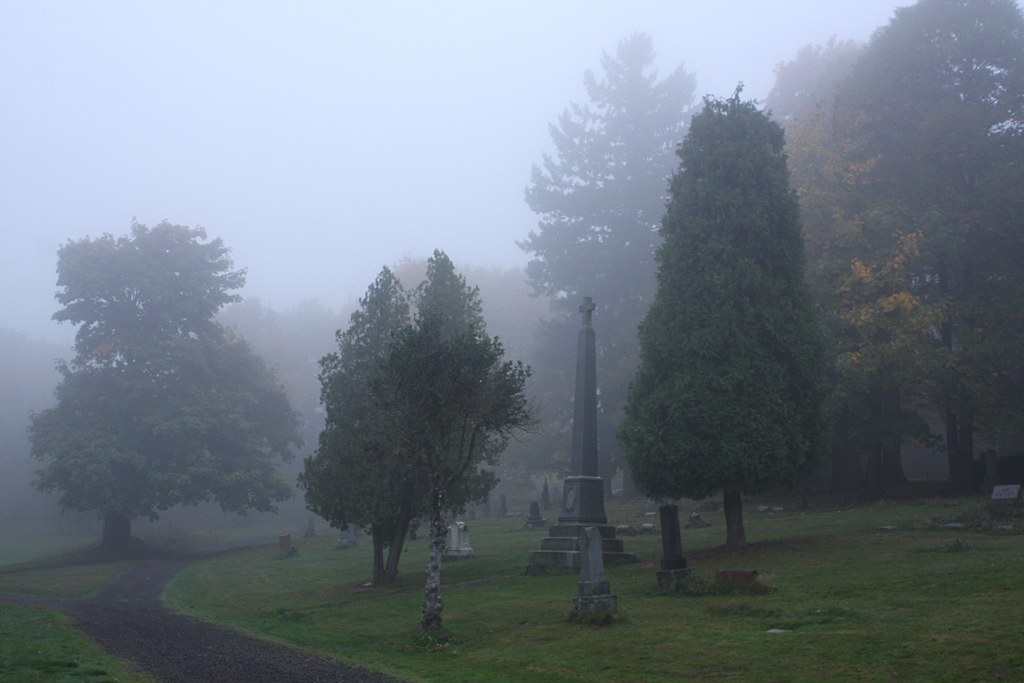The image is a color photograph of a cemetery enveloped in heavy fog, taken during the day. The dense fog warps the scenery, obscuring the horizon and enshrouding numerous trees that tower over the scene. Prominently featured in the middle of the image is a concrete memorial resembling a tower, topped with a cross. In the foreground, a curving walkway begins at the bottom left, flanked by trees on both sides and leading into the background. Scattered throughout the scene are several older tombstones, adding to the somber atmosphere. One particularly tall and vibrant green tree stands on the far right. The image is devoid of people, animals, writing, buildings, or any vehicles, emphasizing the stillness and solitude of this foggy graveyard.